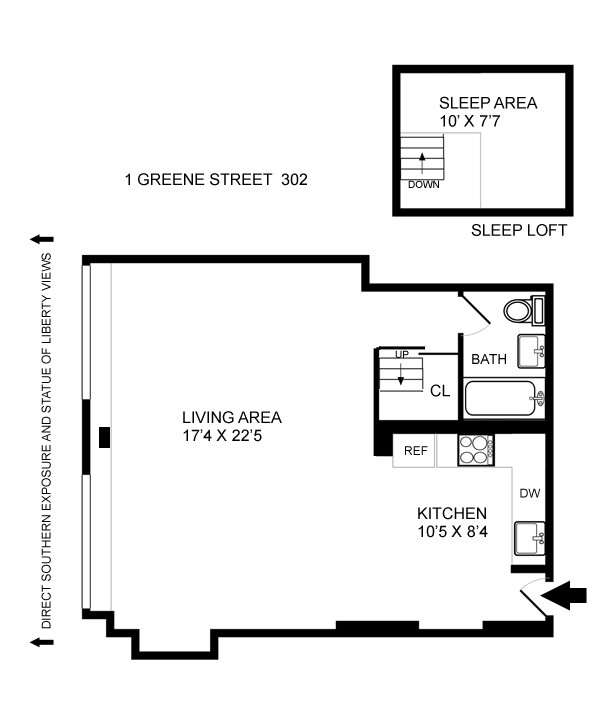This detailed floor plan depicts a modern, two-storey apartment located at 1 Green Street, Unit 302. The layout is presented on a completely white background. 

The central part of the floor plan is a large, square-shaped area. The right half of this space is designated as the living area, measuring approximately 17 feet 4 inches by 22 feet 5 inches. The living area is spacious, ideal for lounging, socializing, and accommodating entertainment needs. 

To the top right of the living area, a bathroom is conveniently situated. Just below, on the bottom right, is the kitchen, which is positioned close to the entryway located on the right side towards the bottom corner of the main square. 

A staircase is located to the left of the bathroom, leading up to an additional sleeping area depicted as a small square at the top right of the main floor plan. This "sleep loft" is accessible via this staircase, marked with a down arrow pointing upwards to indicate the movement direction from the main floor.

Text labels provide additional details: the left-hand side of the floor plan notes the apartment's address, "1 GREEN STREET 302," in capitalized text. On the right-hand side, oriented at a right angle, the text mentions "DIRECT SOUTHERN EXPOSURE AND STATUE OF LIBERTY VIEWS," which is positioned next to a window on the left-hand side of the layout, emphasizing the impressive and desirable vistas available from this unit.